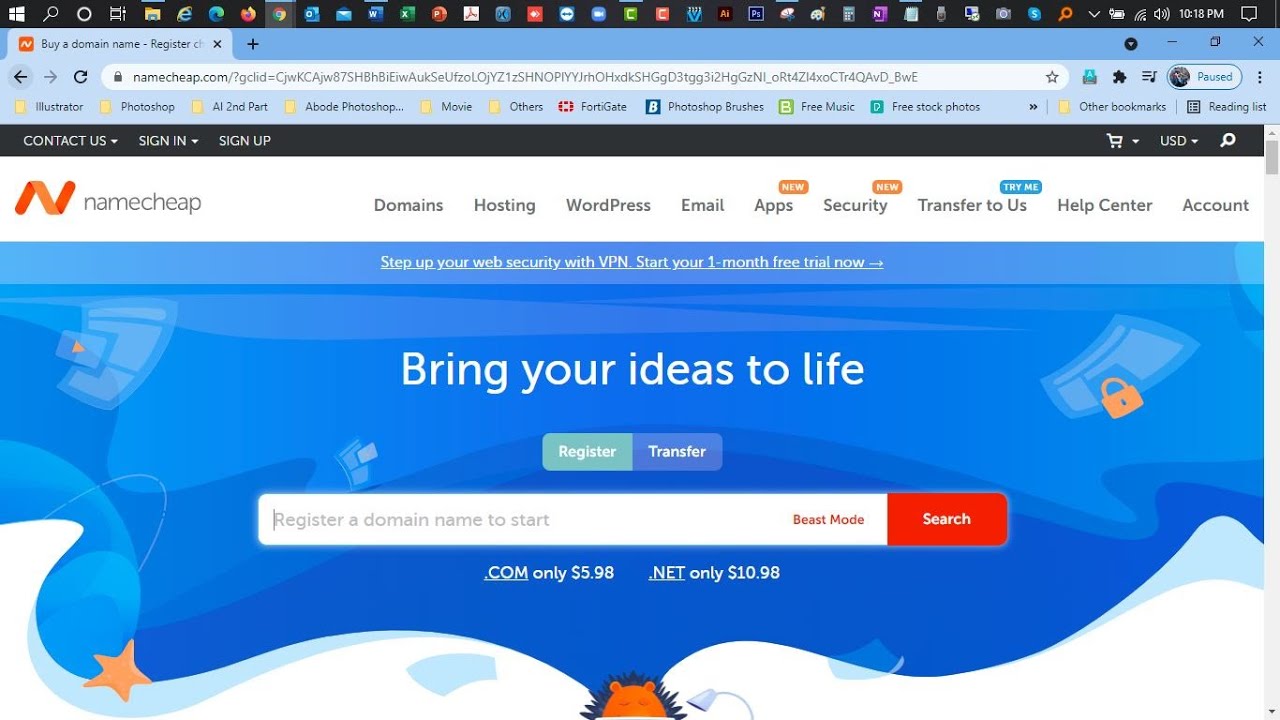This image is a detailed screenshot of a computer screen displaying a webpage. At the very top, there's a black horizontal bar filled with a variety of colorful icons. The area above the bar is blue. On the left side of the screen, there's an open tab that contains black text. Directly below this tab is a search bar. Below the search bar, a row of icons and folders is lined up horizontally. A thick black horizontal line runs across the screen, creating a division.

In the upper left corner, there's a prominent large capital red "N". Next to it, in lowercase gray letters, reads "Name Cheap". To the right of this logo, there is a navigation menu containing the following links: Domains, Hosting, WordPress, Email, Apps, Security, Transfer to Us, Help Center, and Account.

Below the navigation menu, the background is blue, featuring a central white text that reads, "Bring Your Ideas to Life." Approximately two rows below this central text, there are two touching rectangles. The rectangle on the left is green with white text that reads "Register", while the one on the right is blue with white text that reads "Transfer". Further below, there is a search bar with placeholder text in gray that says, "Register a Domain Name to Start".

This screenshot captures the interface and layout of a webpage, likely related to domain registration and hosting services.